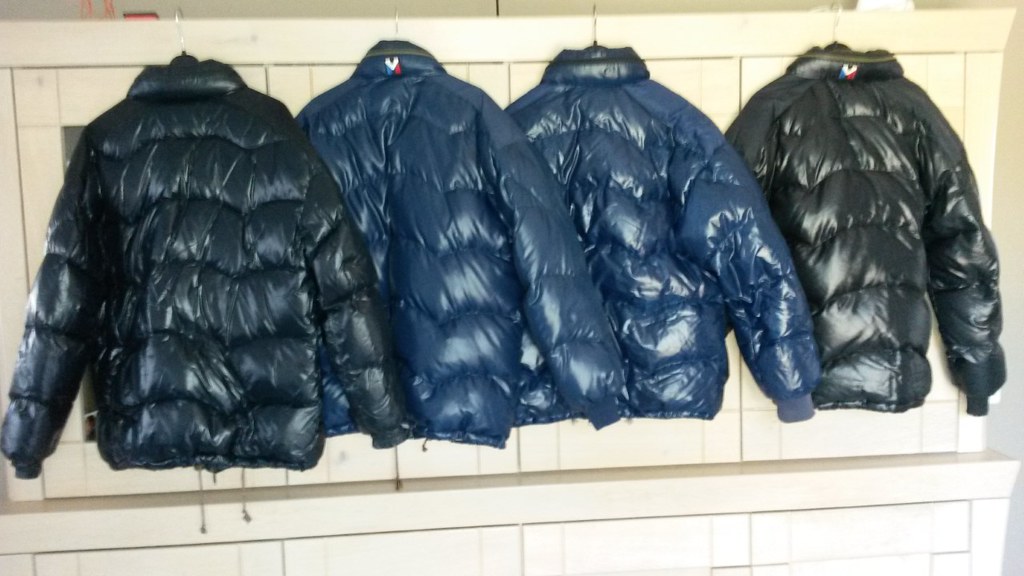This horizontally cropped photograph captures the backs of four quilted, puffy winter jackets hanging against a tiered white background with subtle perpendicular lines. Despite the slightly yellow tint and low quality, the image distinctly highlights the puffiness and glossy texture of the jackets. Arranged from left to right, the jackets include a dark blue jacket on the far left, two medium blue jackets in the center, and a nearly black or dark blue jacket on the right. Two of the jackets, specifically one in the center and the one on the right, feature a white "V" on the back of their collars with a stripe in the colors of the Mexican flag – green and red – running down from the "V". The photograph captures the depth and texture of the jackets through the careful shading and lighting, with visible overlapping sleeves enhancing their puffy appearance.